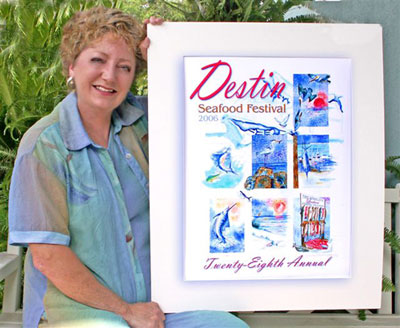The image showcases a woman seated on the left side of the frame on a white wooden bench. She is positioned in front of vibrant green-leaved trees, adding a lively touch to the setting. The woman holds a sign advertising the Destin Seafood Festival from 2006. The sign features several illustrated depictions of dolphins and various fish swimming harmoniously in the ocean. At the bottom of the sign, "28th annual" is written in pink cursive lettering.

The woman is dressed in a short-sleeved, button-up shirt displaying a gradient of medium blue, light blue, and orange hues. Underneath, she wears a light blue t-shirt paired with matching light blue jeans. She has short blonde hair and engages warmly with the camera, smiling brightly at the photographer.